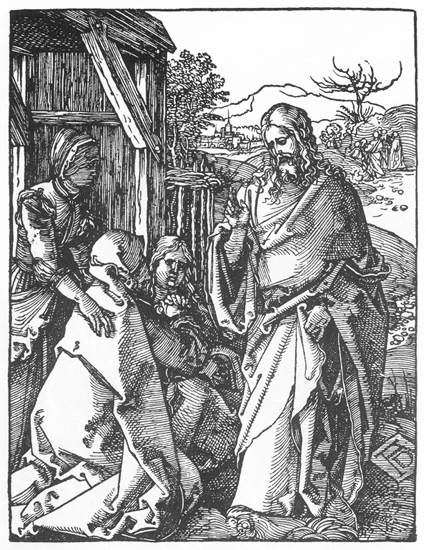The image is a highly detailed, black and white pen and ink drawing, reminiscent of an ancient etching. It portrays a biblical scene with a person who appears to be Jesus, standing prominently in the foreground. He is depicted with long hair, a beard, and a mustache, and is dressed in traditional biblical robes. To his left, two women are kneeling, one with a blanket over her head, embodying solemn expressions. Behind them, a third woman stands, dressed in a dress with a bonnet and ruffled sleeves, her arm resting on one kneeling woman's shoulder. The setting is outdoors, featuring a wooden structure such as a porch or a manger with sparse vegetation including trees that resemble Joshua trees. In the distant background, a cityscape and mountains are faintly visible, adding depth to the scene. The overall composition suggests a religious narrative captured in meticulous detail.